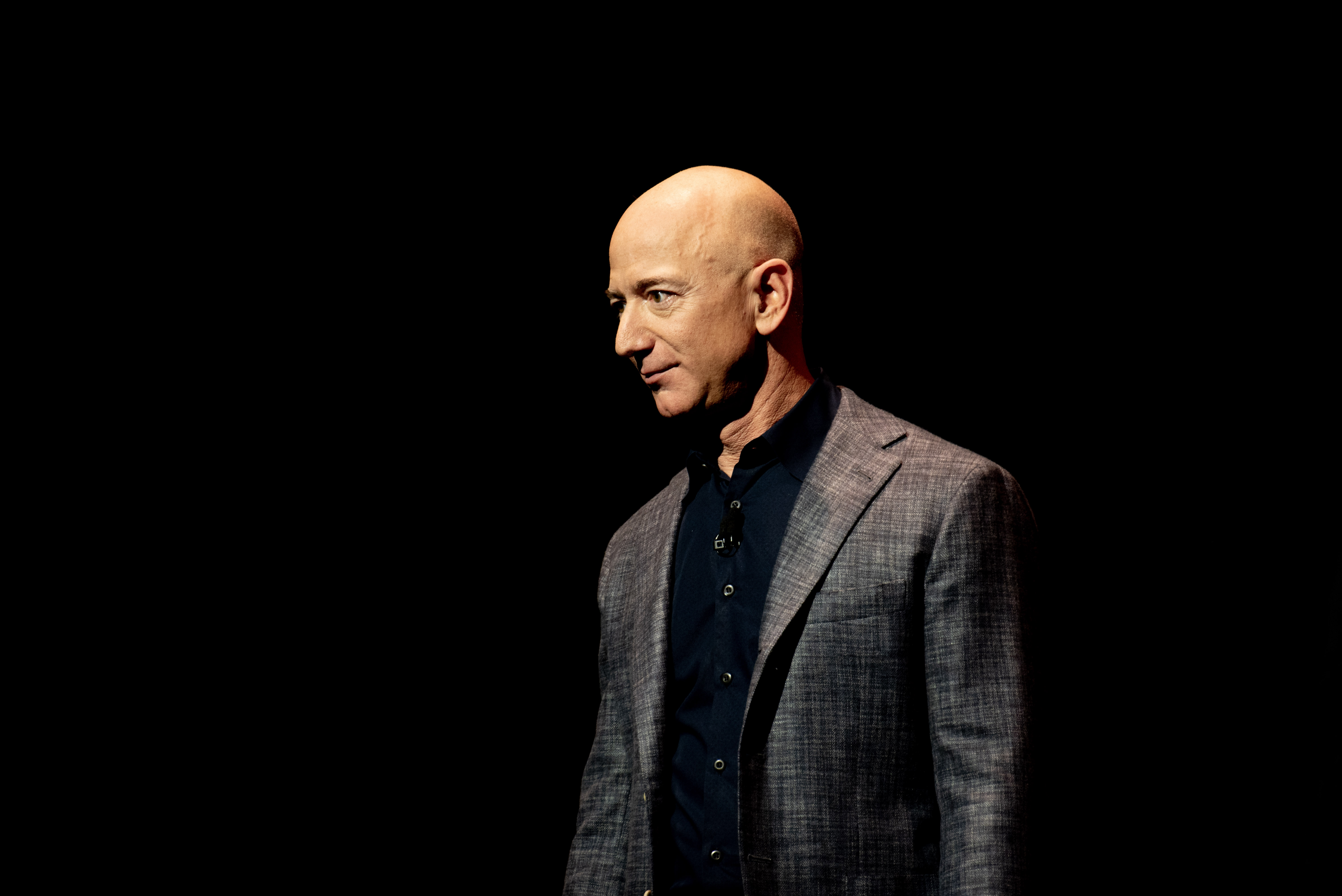The photograph features Jeff Bezos, captured indoors with a pitch-black background that starkly separates him from the setting. The image is wider than it is tall, measuring approximately six inches wide by four inches tall, emphasizing a rectangular shape. Bezos, an older Caucasian man, is prominently displayed from the waist up, slightly off-center to the right. He is bald but with a small amount of hair behind his ear. His posture is slightly turned to the left, allowing most of his torso to be visible, while his head tilts downward with a neutral expression, as if he might be giving a presentation or speech. Shadows beneath his chin suggest the lighting is directed from above. He is dressed in a distinguished outfit consisting of a silver-gray striped dress jacket over a navy blue button-up shirt. A small microphone is clipped to the center of his shirt, indicating that he might be addressing an audience. His mouth is closed, and his hands rest by his sides, enhancing the formal and composed demeanor of the scene.